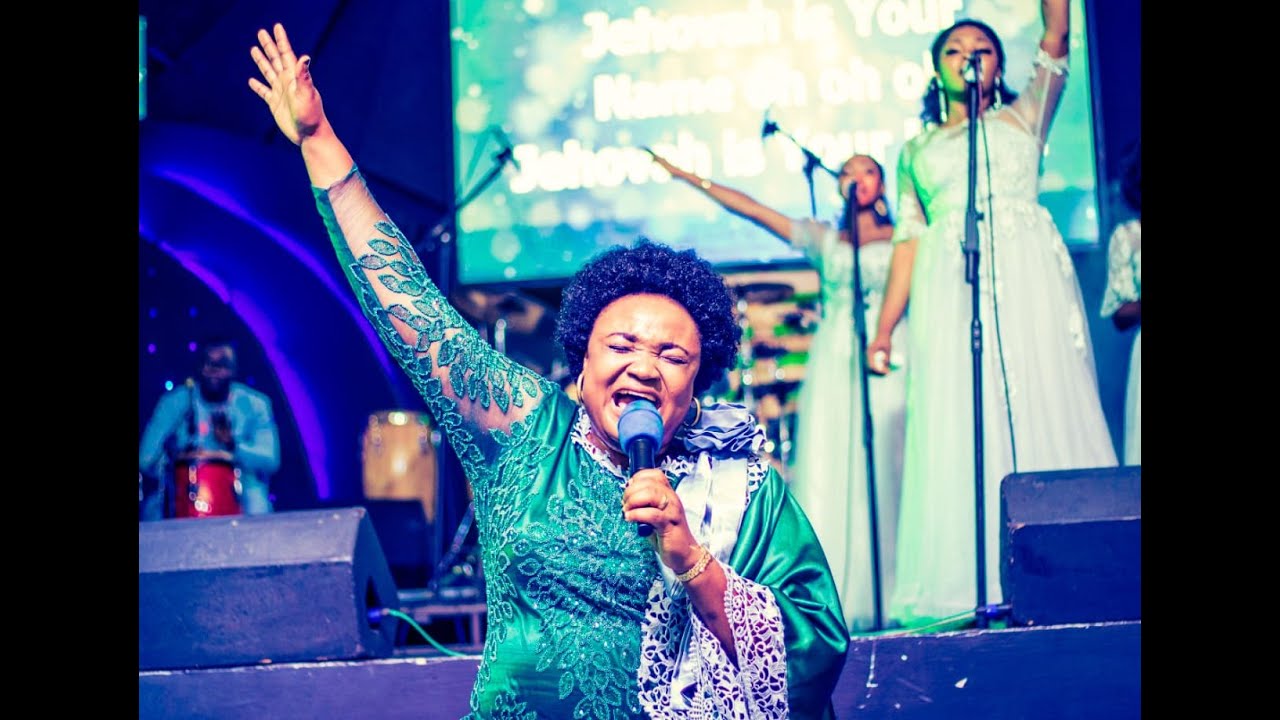This image captures a vibrant concert scene focused on an African-American female singer standing at the front of a stage with closed eyes, deeply immersed in her performance. She is holding a microphone in her left hand and raising her right arm, fingers spread apart. She has short, curly afro hair and wears a green dress featuring floral designs, a see-through sleeve revealing part of her arm, and a white shawl hanging over her shoulder. She also sports two large gold earrings. 

To her right, three younger African-American women appear, possibly her backup singers. They have black hair, with at least one wearing pigtails, and are all dressed in white dresses. Each backup singer holds a microphone and mimics the lead singer's pose, with arms raised—one directly upwards and another slightly outward. 

In the background, the stage is set against a dark blue backdrop with a video board displaying song lyrics in white text. Towards the left and near the bottom of the frame, a man in a light-colored, long-sleeved suit jacket plays a red bongo drum. The audience, although partially obscured, can be seen seated and watching attentively. The blue hues dominate the scene, adding to the concert’s atmospheric lighting. This detailed tableau captures the energy and coordination of a passionate live performance.